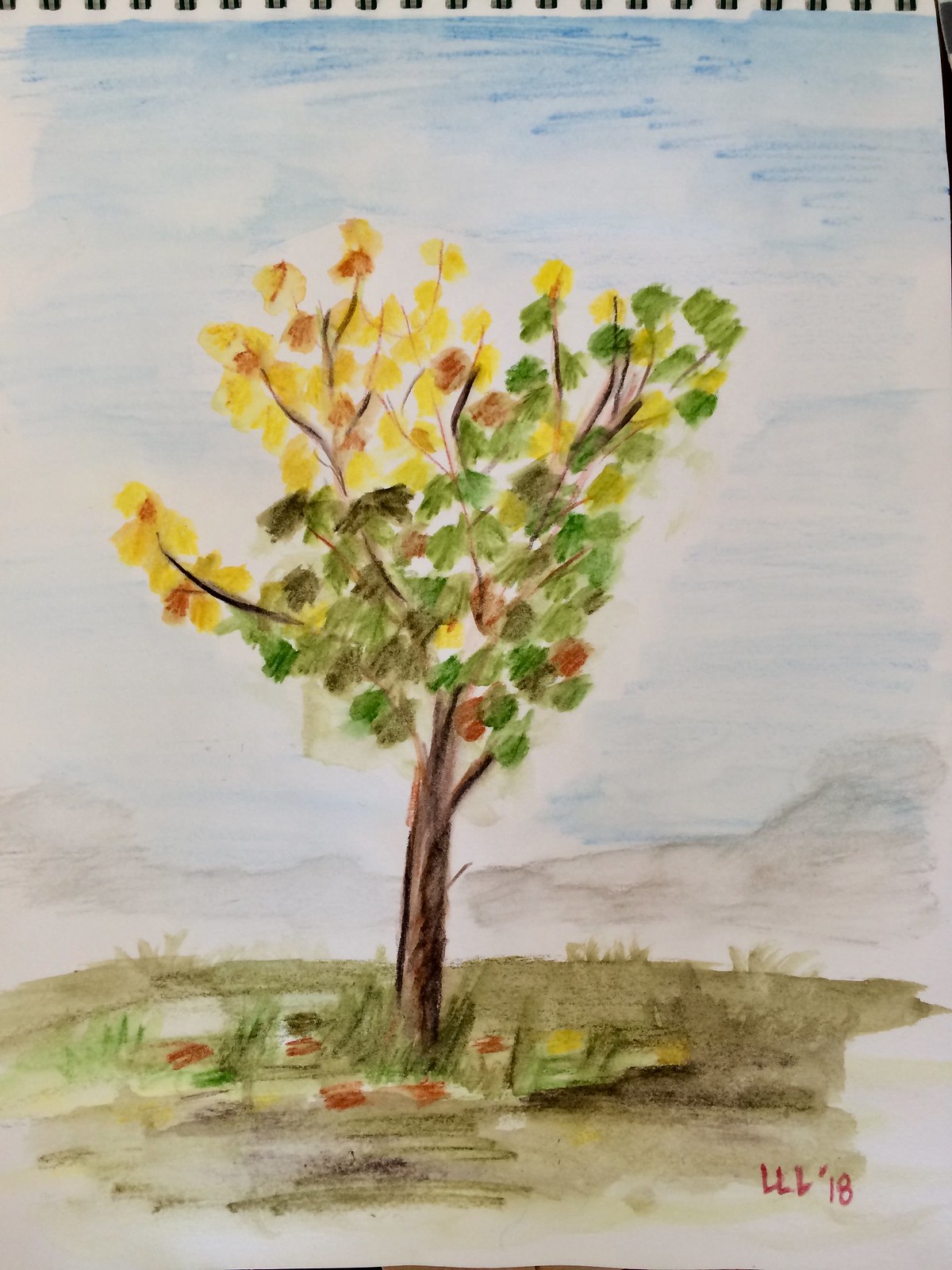This image showcases a meticulously captured photograph of an art piece rendered in a notebook. The artwork appears to be created using watercolor pencils, masterfully blending the hues of traditional colored pencils with the fluidity of watercolors. The subject of the illustration is a solitary tree, its canopy adorned with a mix of green, yellow, and brownish-orange leaves, suggesting the transition of seasons. The tree is rooted in a grassy, slightly muddy terrain, with a subtle touch of a pale blue sky peeking through the background, lending a serene atmosphere to the scene. In the bottom right-hand corner, the artist has signed the piece with the initials "L.L.L." and the year "18," adding a personal touch to this charming depiction of nature.